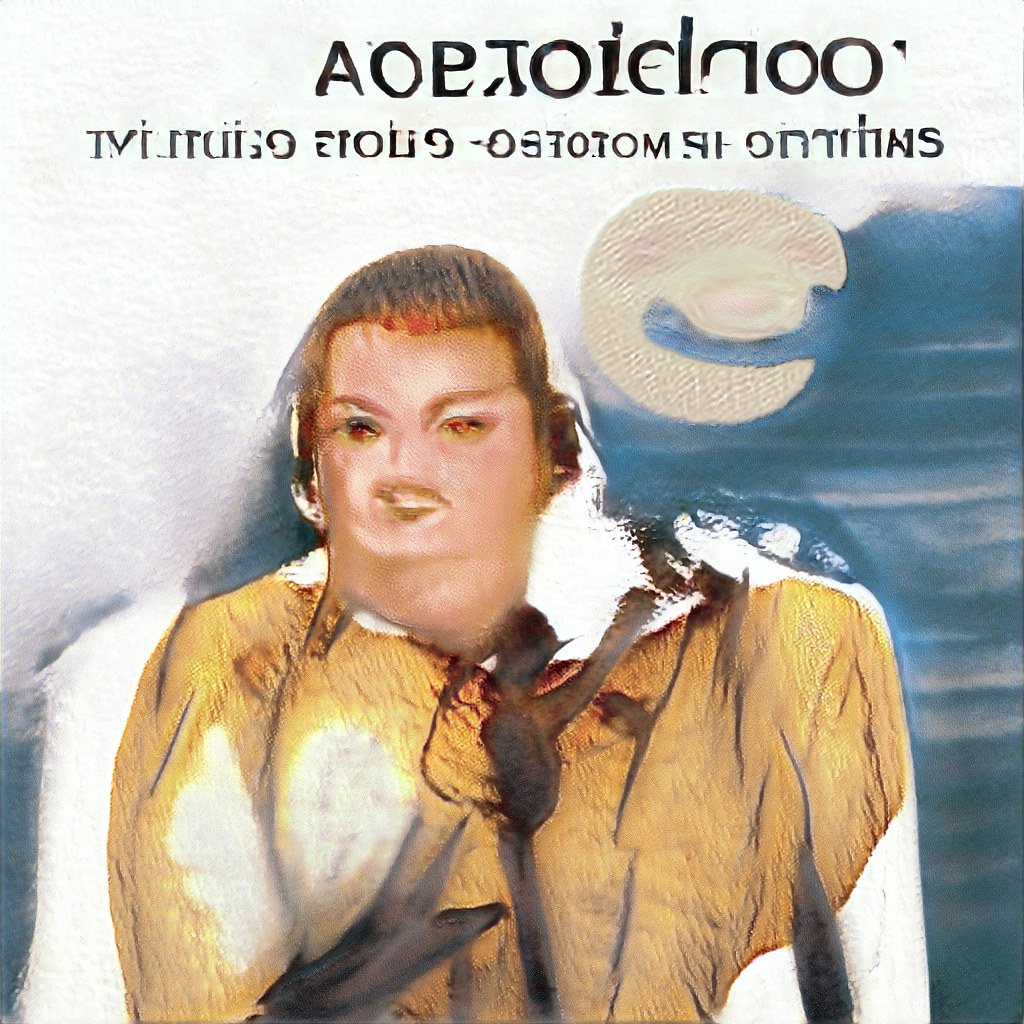This "artsy" and somewhat "creepy" image appears to be AI-generated, featuring a human face with short brown hair and distinct facial features. The subject has red eyes, big eyebrows, and dark brown lips that may suggest a slight smile, though the nose is barely visible. The background is divided diagonally into two main colors: dark blue on the right side and white on the top left. At the top of the image, there's some illegible black text in a strange font, possibly written backwards or in an unfamiliar language, adding to the eerie effect. The person appears to be wearing a brownish-white shirt. Additionally, in the top right corner, there's an ambiguous celestial object—perhaps a sun or a moon—with a blue line running through it. The overall impression is the face's unsettling, almost "clutch cargo" quality, where the mouth seems out of place, reminiscent of the mid-20th-century animation technique.